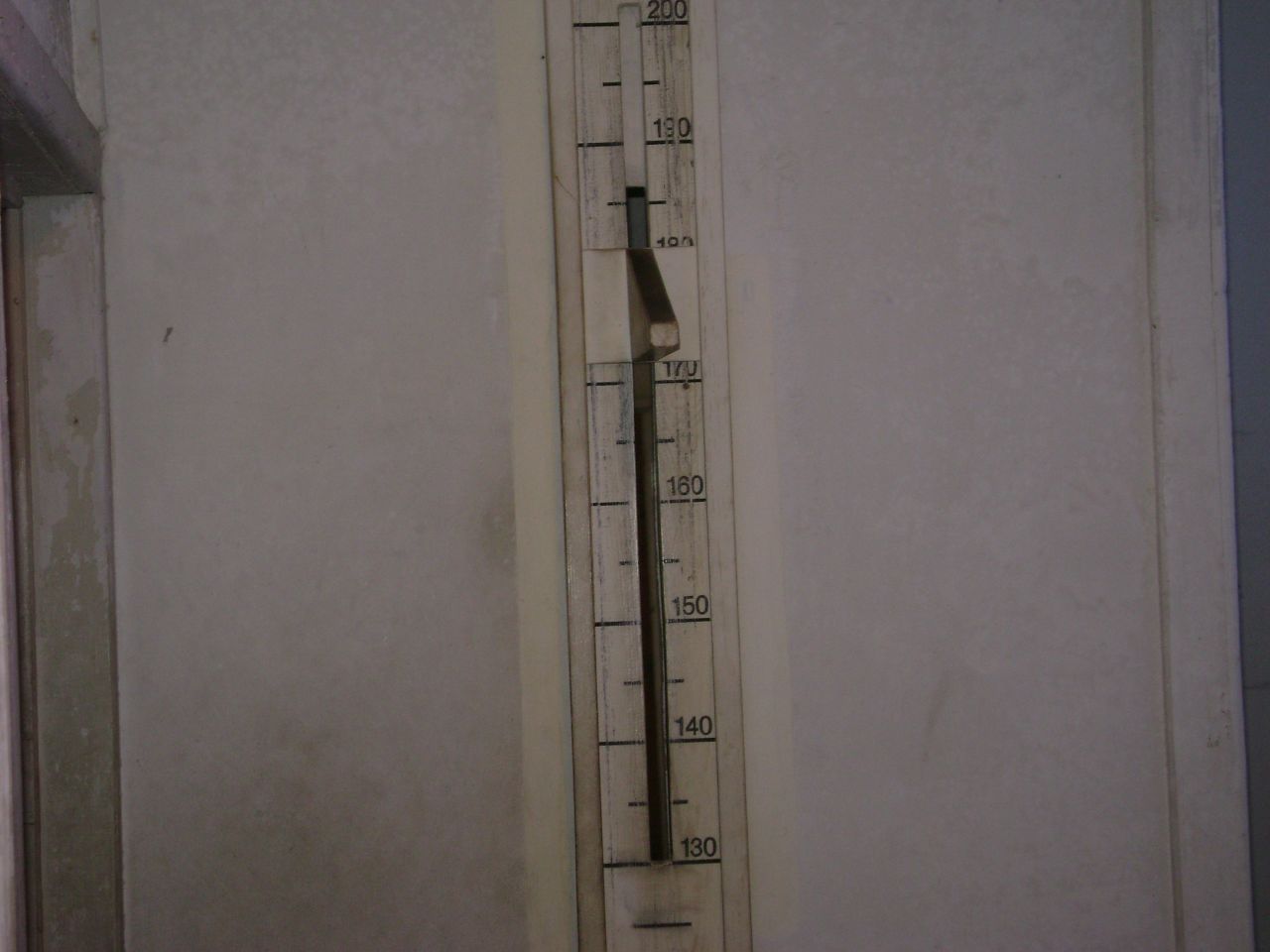The image depicts a vintage mercury thermometer mounted on a white wall. The thermometer, designed in an old-school style, features a white casing and a clear glass tube filled with mercury in its center. The thermometer is affixed to a vertical rectangular ruler-like grid, marked with alternating short and long horizontal dashes that are numerically labeled. This grid serves as the scale for temperature measurement. The thermometer is held in place by a small metal bar at its upper section. On the left edge of the photo, white vertical crown molding frames the scene, possibly indicating the border of a bookshelf or a doorway, while similar molding appears on the right edge. The overall composition highlights the antique design and intricate details of the thermometer against the simplicity of the white wall and moldings.